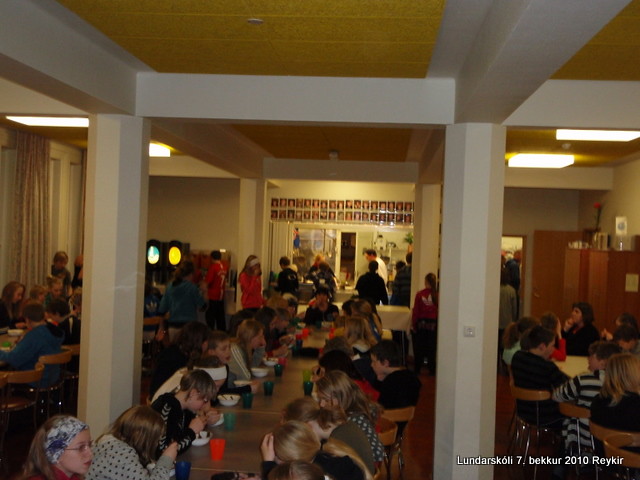The photograph titled "Lunderskolli 7, Becker 2010, Raker" captures an interior scene of a lively room filled with young pre-teens seated at three long, brown-chaired tables, suggesting a cafeteria setting that's slightly more refined due to the presence of floor-to-ceiling white columns. These young Caucasian children, each with small white bowls in front of them, appear to be eating pasta, indicating a shared meal experience. The setting is likely a party or community gathering. The room features a yellow ceiling and white beams, with various colored glasses - green, red, and blue - scattered on the tables, adding to the vibrant ambiance. In the background, a low-resolution kitchen area can be seen, where children line up with trays, waiting for their turn to pick up food from a window. There are also cupboards resembling office furniture to the right, and a distinctive blue and yellow oval light fixture to the left, subtly enhancing the space's decor. Additional details include a row of indistinct photographs hanging on the back wall and a drink station, hinting at a venue designed for communal dining and social interaction.